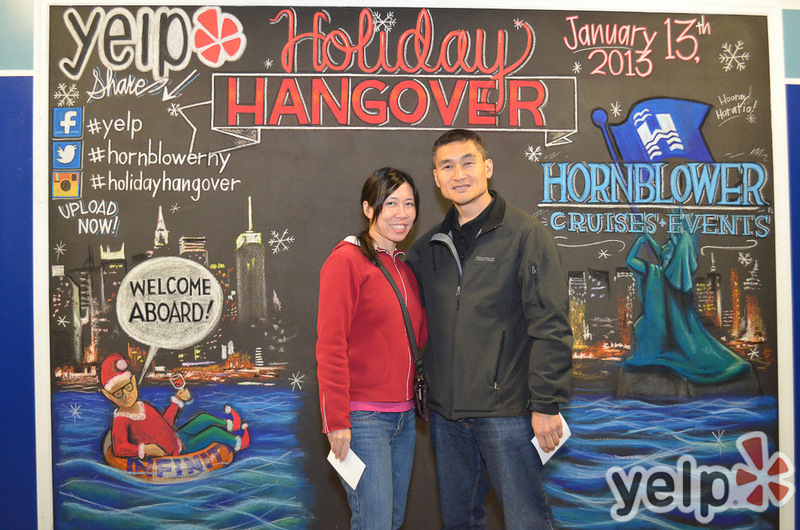This detailed color photograph, taken in landscape orientation, features an Asian couple standing side by side near the bottom center of the image, depicted from their heads to their knees. The man, taller than the woman, wears a black windbreaker over a black golf shirt paired with blue jeans, and holds a white note card in his left hand. The woman, to his left, dons a red sweatshirt, blue jeans, and a black cross-body purse. She also holds a white note card in her right hand. Neither of them wears glasses.

The backdrop is a large poster wall with a chalkboard-like design. This background prominently features the event title "Holiday Hangover" in red script chalk handwriting, along with the date, January 13th, 2013, in the top right-hand corner. At the bottom right corner, the Yelp logo and name are displayed. To the right side of the couple is the Hornblower Cruises and Events logo, depicted with a blue flag featuring a white "H." Additionally, there's a graphic of a blue figure blowing a horn amid a nighttime city skyline and a bay, creating an oceanic motif across the lower third of the image.

A charming illustration of a Christmas elf dressed in a Santa suit, floating in an inner tube, adds a festive touch. The elf holds up a drink and is accompanied by a conversation cloud that reads, "Welcome Aboard!" The overall setting, enhanced by the city skyline and river motifs, provides a scenic bay view that adds depth and context to this celebratory event capture.